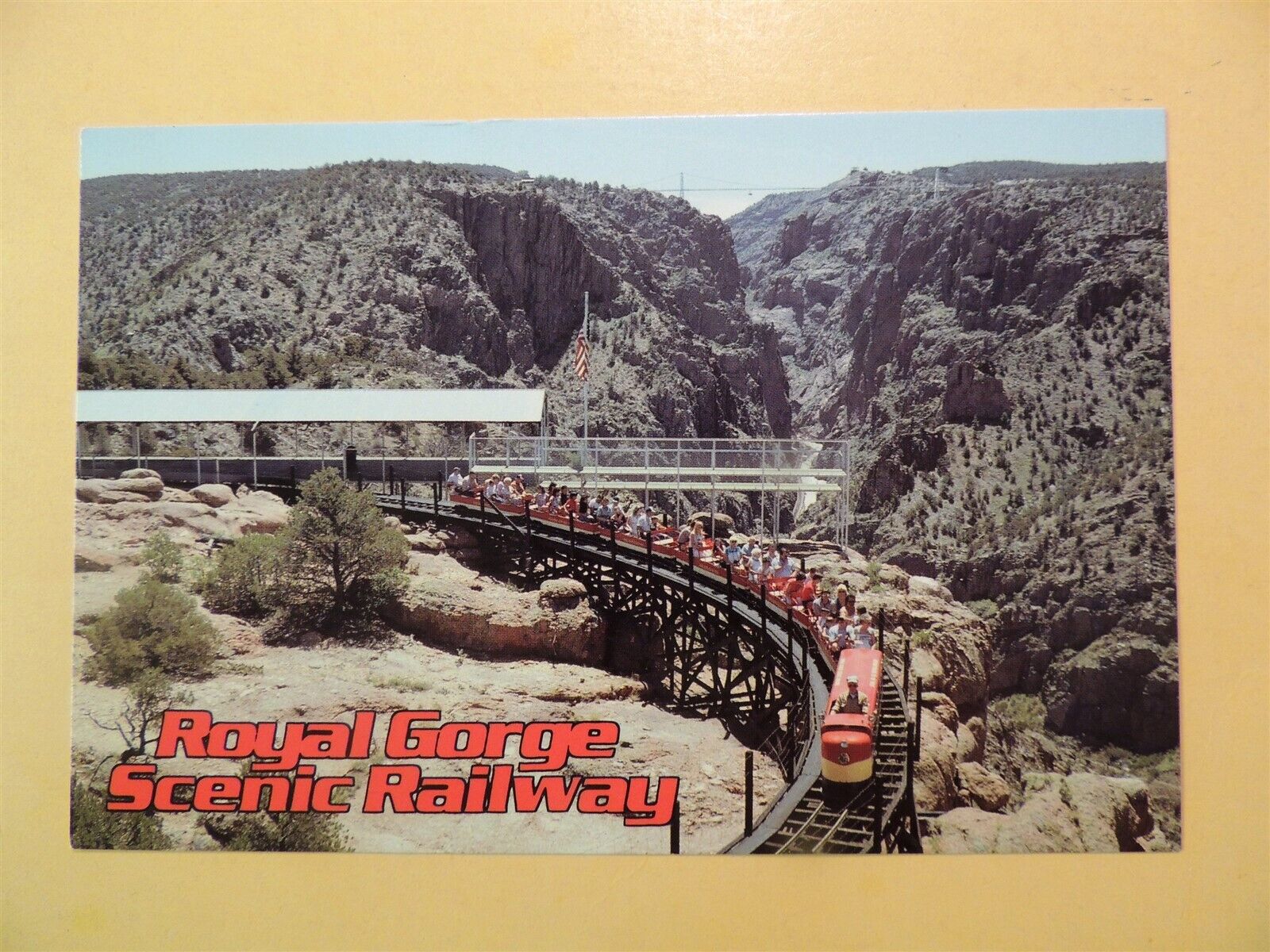The image is a postcard-style horizontal photograph of the Royal Gorge Scenic Railway, set on a cream-colored background. The writing "Royal Gorge Scenic Railway" appears in reddish-orange at the bottom left. The scene features a rugged, desert-like landscape with rocky mountains and sparse grass, indicating a remote wilderness area. Central to the image is a small tourist train painted in orange and yellow, with a black track curving from the bottom left towards the center. The train has about ten cars filled with people and is led by a conductor visible in the front. The track, elevated on short stilts, leads to a silver-roofed exit port with open walls and an observation platform extending over a gully. An American flag is seen in the background, enhancing the scene's picturesque, postcard-worthy appeal on a clear day.